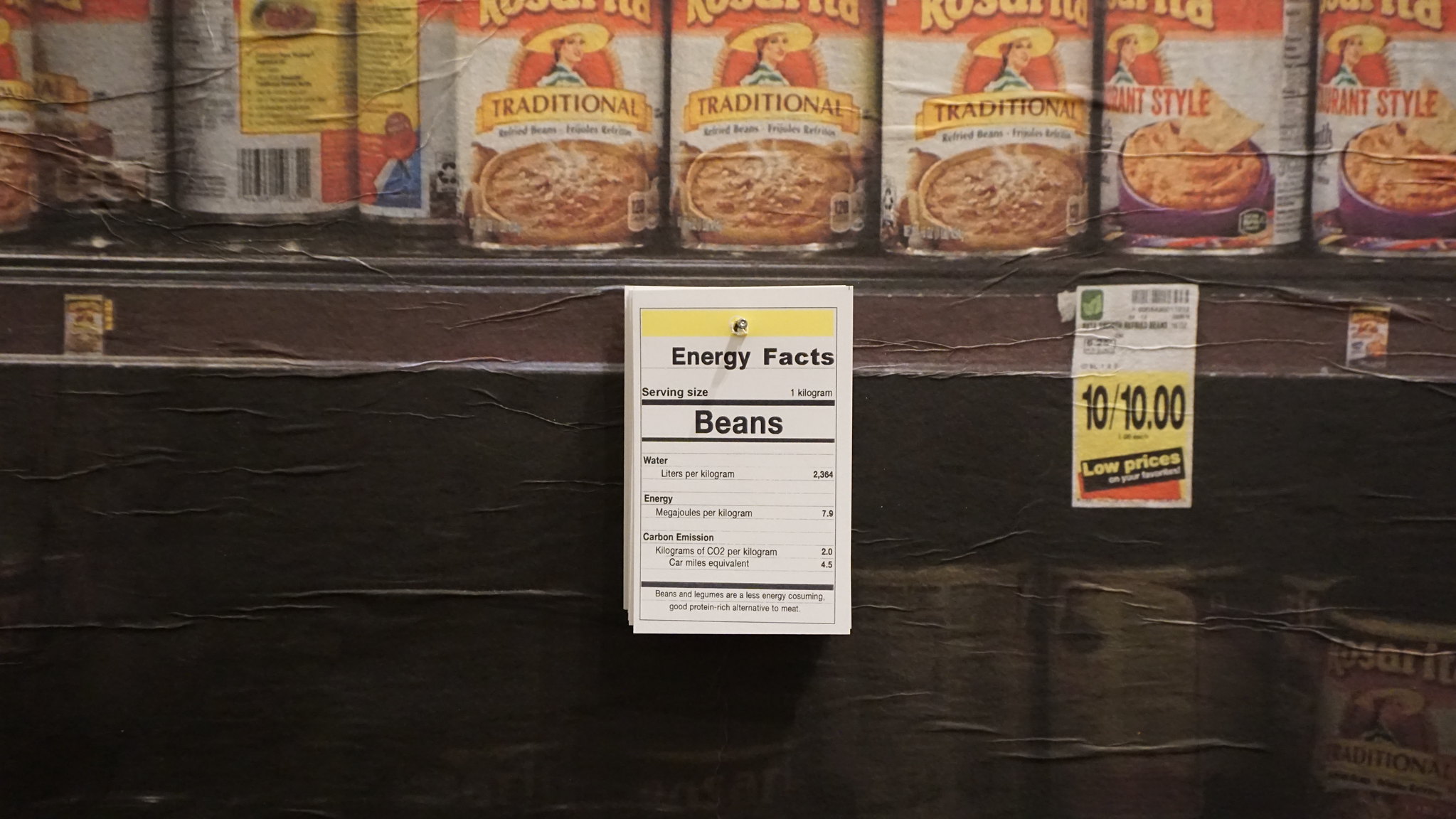This detailed photograph depicts a grocery store shelf, with the focus on an assortment of canned goods branded under the Rosario Traditional label. The cans, featuring a striking logo of a woman in a green and white top with a large yellow hat, are neatly arranged on a top shelf. The labels are notable for their white and red color scheme, with "Traditional" displayed on a yellow banner with brown lettering, while "Restaurant Style" is in red letters. In total, five cans are clearly visible, with three labeled "Traditional" and two labeled "Restaurant Style." Additionally, there are several other cans partially obscured. 

The shelf display includes various signage: a white piece of paper with a yellow border at the top and a black frame containing black text that reads "Energy Facts Beans," detailing nutritional information, and a prominent price tag announcing "10 for $10" in white and yellow, promising low prices to shoppers. The image quality is affected by noticeable wrinkle marks, suggesting it is a photograph of an older photograph.